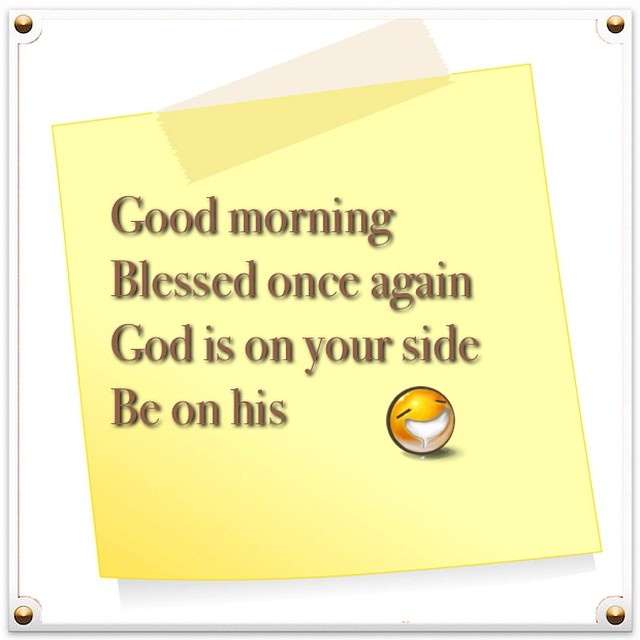The image is a digitally illustrated clip art of a yellow sticky note, appearing to be taped to a white background with a piece of clear tape at the top, placed diagonally. The sticky note features a silver-white border with rivets in each corner, giving it the appearance of being framed. In brown text, the note reads: "Good morning. Blessed once again. God is on your side. Be on his." Below the text, there is a small emoji with a wide, drooling grin and closed eyes. The emoji has an orange-yellow tint and is slightly tilted. The drool extends from its smile, and it casts a subtle shadow onto the sticky note.